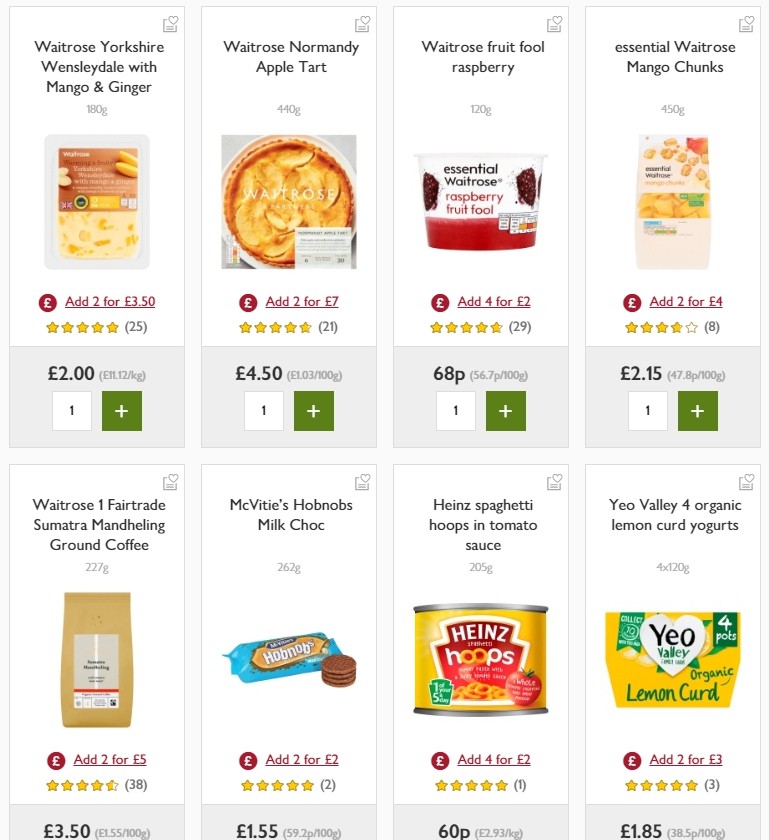This image is a detailed screenshot of a shopping website featuring eight different items available for purchase in British Pound Sterling. The items are listed as follows:

1. **Waitrose Yorkshire Wensleydale with Mango and Ginger**
2. **Waitrose Normandy Apple Tart**
3. **Waitrose Fruit Full Raspberry**
4. **Essential Waitrose Mango Chunks**
5. **Waitrose One Fairtrade Sumatra Mandheling Ground Coffee**
6. **McVitie's Hobnobs Milk Chocolate**
7. **Heinz Spaghetti Hoops in Tomato Sauce**
8. **Yeo Valley Organic Lemon Curd Yogurts**

Each product listing includes the following details:
- The **name of the item** prominently displayed.
- The **weight** of the product located underneath the name.
- A **picture** of the item for visual reference.
- A **pound symbol** indicating that an additional 2 or 4 items could be purchased for a discount.
- A **rating system** showing customer reviews.
- The **price** in British Pound Sterling.
- The **quantity** of the item currently added to the shopping cart.

This comprehensive display aims to provide shoppers with all the necessary information required to make informed purchasing decisions.